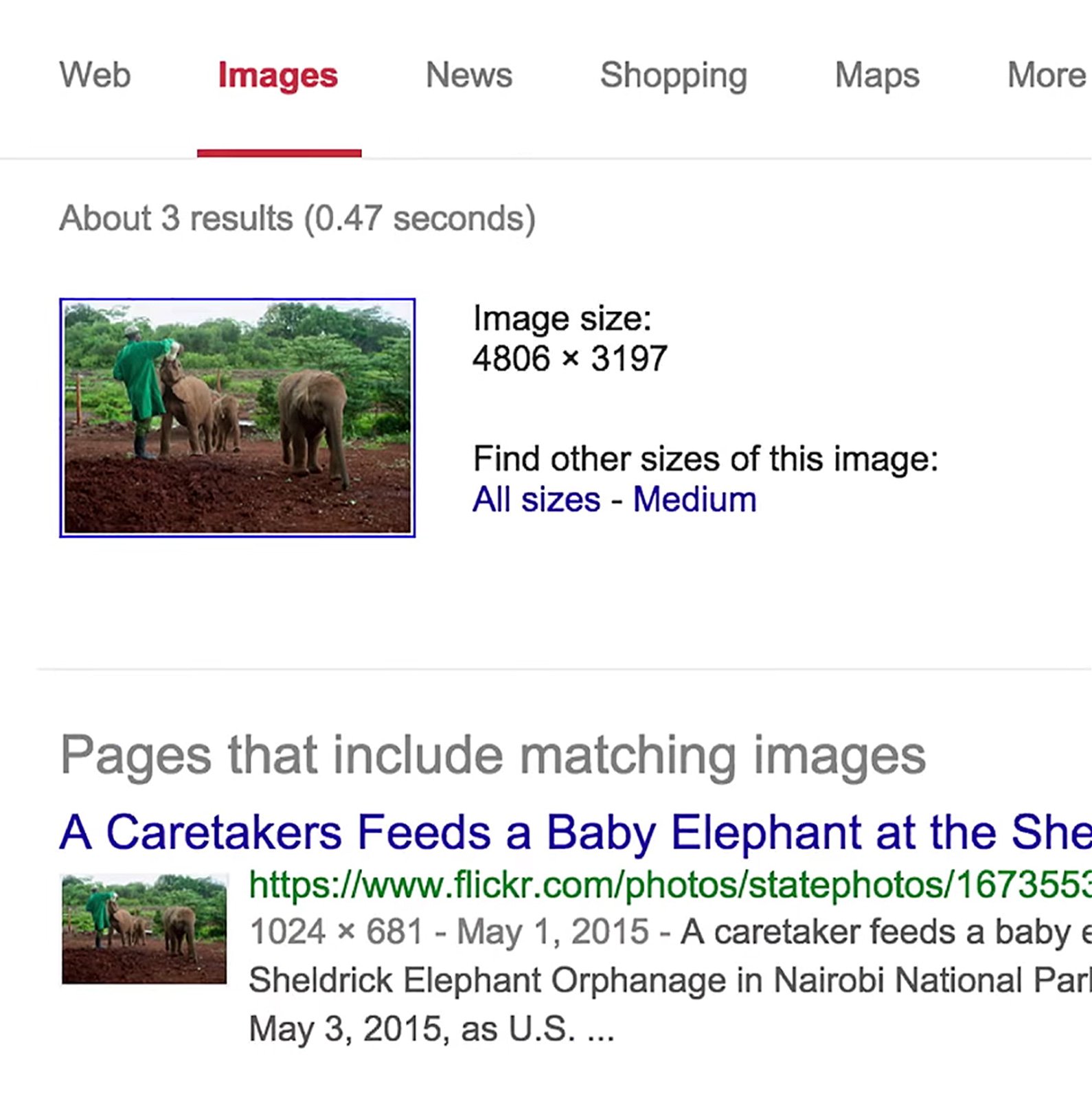The image depicts a Google search results page with a white background. The options "Web," "Images," "News," "Shopping," "Maps," and "More" are listed at the top, with "Images" highlighted in red and underlined, while the other options are underlined in gray. Below, the search results indicate approximately three results found in 0.47 seconds. 

An image is displayed featuring a couple of young elephants standing on a dirt patch surrounded by trees. A man, possibly a caretaker, is standing next to them. The image is noted for its resolution of 4806 by 3197 pixels. Below the image, there is an option to find other sizes of the image, marked as "all sizes," with a gray underline. Further down, a section titled "Pages that include matching images" features the same picture and text indicating "A caretaker feeds the baby elephant at the SHE," followed by a URL. The reduced size of the image, 1024 by 681 pixels, is also mentioned.